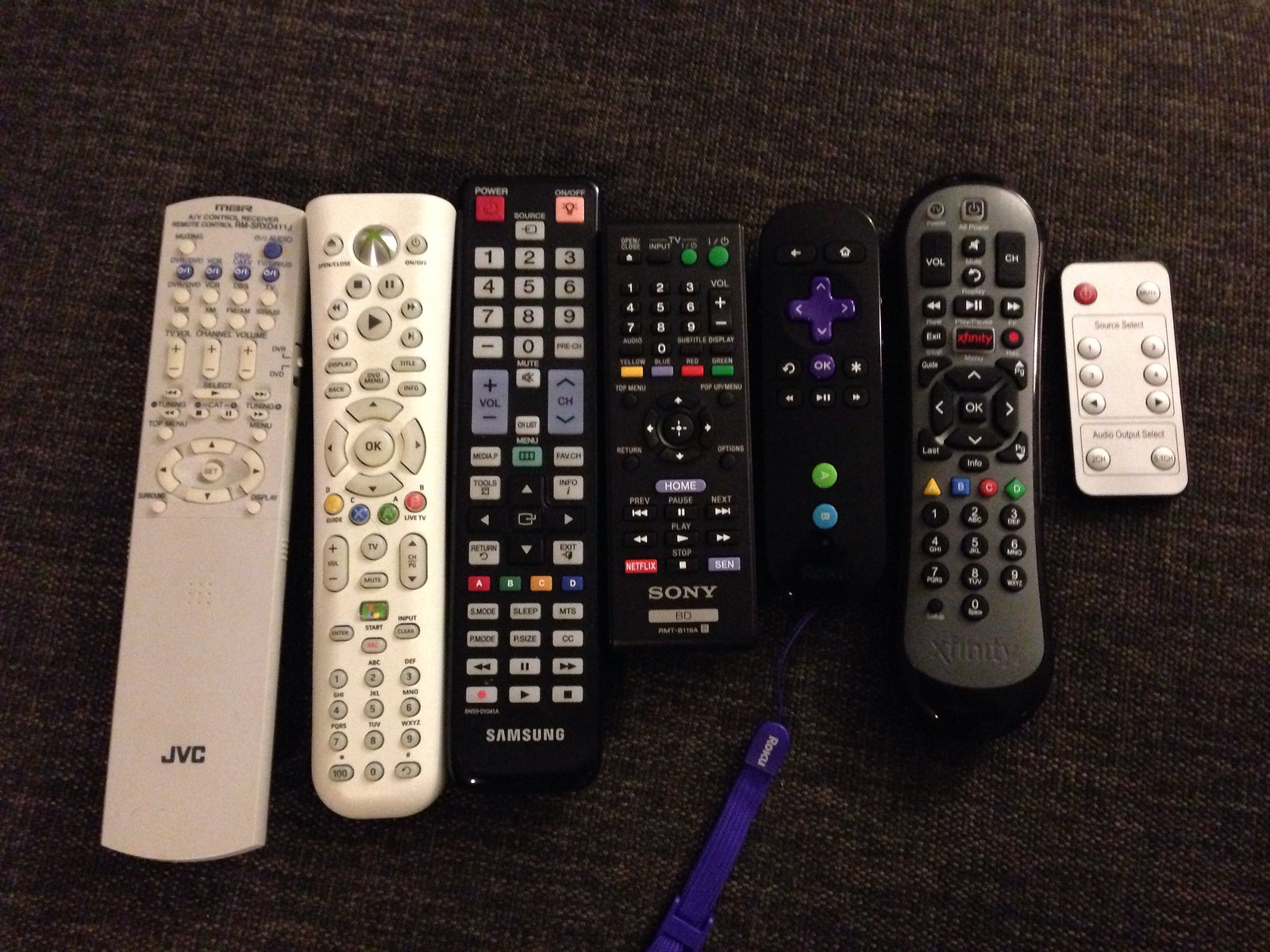This is a detailed color photograph of seven remote controls neatly lined up side by side on a heathered maroon and tan fabric, possibly upholstery or a short nap carpet. The remotes vary in size, brand, and color, arranged from left to right in descending order of size, with one exception.

1. **Far Left**: A long silver remote with the brand "JVC" at the bottom, featuring white and light blue buttons.
2. **Second from Left**: An elongated wedge-shaped white remote with opaque buttons and no visible brand name.
3. **Third from Left**: A black Samsung remote with a mix of white, red, pink, blue, and several other colored buttons, including A, B, C, and D buttons.
4. **Fourth from Left**: A black Sony remote, smaller than the Samsung remote, with colorful buttons including two round green ones and a row of yellow, gray, red, and green buttons.
5. **Third from Right**: A small black remote with a wrist strap and minimal buttons. It has a cross-shaped directional pad in blue with white arrows and two round buttons in lime green and sky blue.
6. **Second from Right**: An Xfinity remote, black with some gray detailing, featuring buttons in various colors including yellow, blue, red, and green.
7. **Far Right**: A very small flat silver remote with about ten light silver buttons and a red power button at the top left, likely for a device like a tower fan or electric fireplace.

The remotes are all in good condition, suggesting they are relatively new. In the foreground, there is a blue pen angled slightly to the right, adding to the composition of the scene.